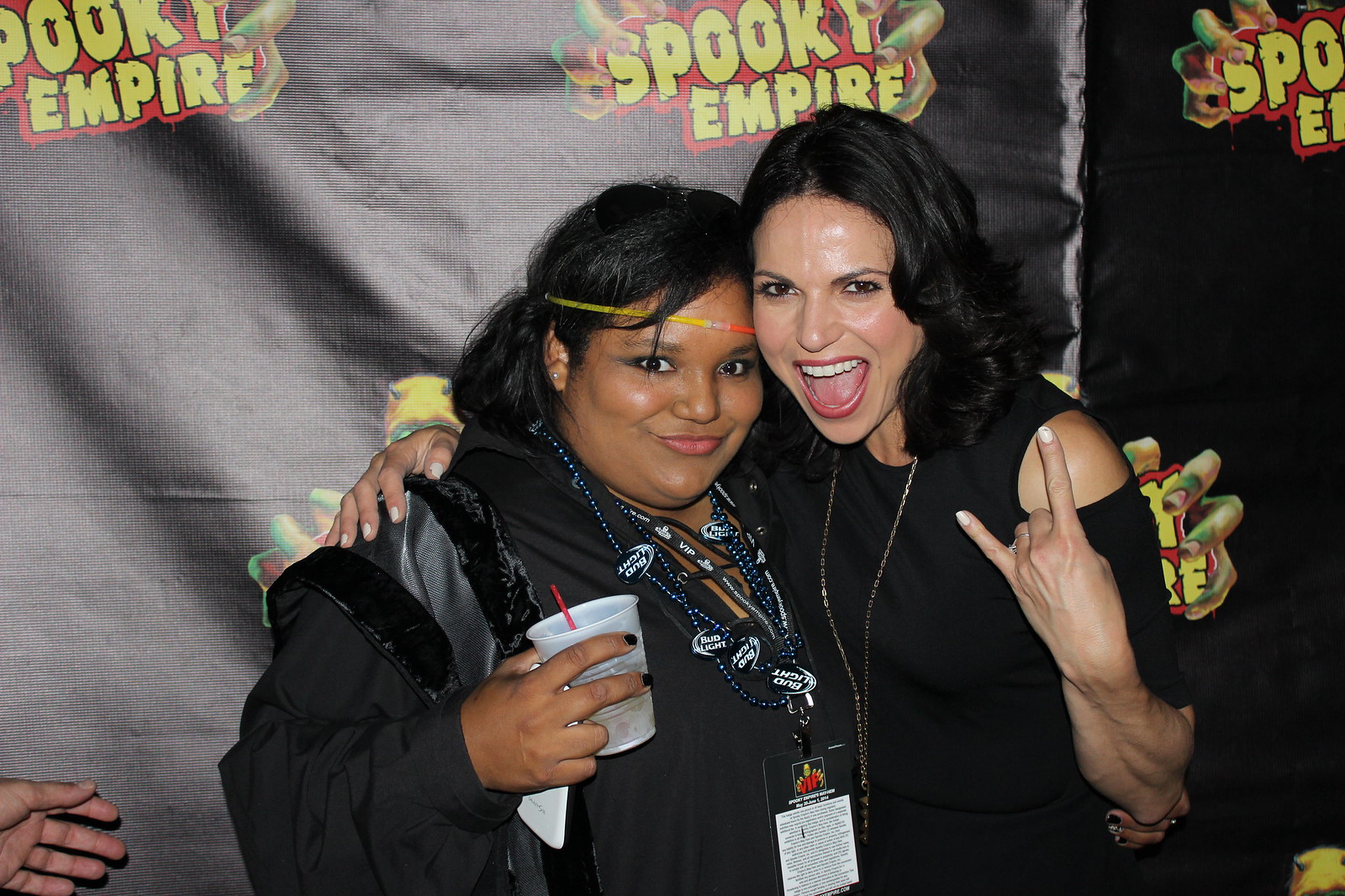In this lively photograph, two women are joyfully celebrating in front of a backdrop that prominently features the "Spooky Empire" logo, repeated several times in yellow text with a red outline. The logo appears in the top left, center, top right, and again behind each woman. 

The woman on the left has caramel skin, possibly indicating Southeast Asian heritage, and is slightly heavier set. She's adorned with Bud Light bead necklaces and wears a glow stick headband. She holds a drink in her left hand and has a lanyard with a badge around her neck. Dressed in all black, she exudes a festive energy.

The woman on the right, who has fairer skin and dark brown hair, stands slightly taller. Her mouth is wide open in a joyous, toothy grin, and she sticks out her tongue while flashing a reversed rock-and-roll hand symbol towards the camera. She is also dressed in black and has her arm around her friend, enhancing the sense of camaraderie and celebration.

The background shows creepy hands emerging towards the women, contributing to the spooky and festive theme of the "Spooky Empire" event. The overall mood is one of excitement and revelry, perfectly capturing the spirit of the occasion.